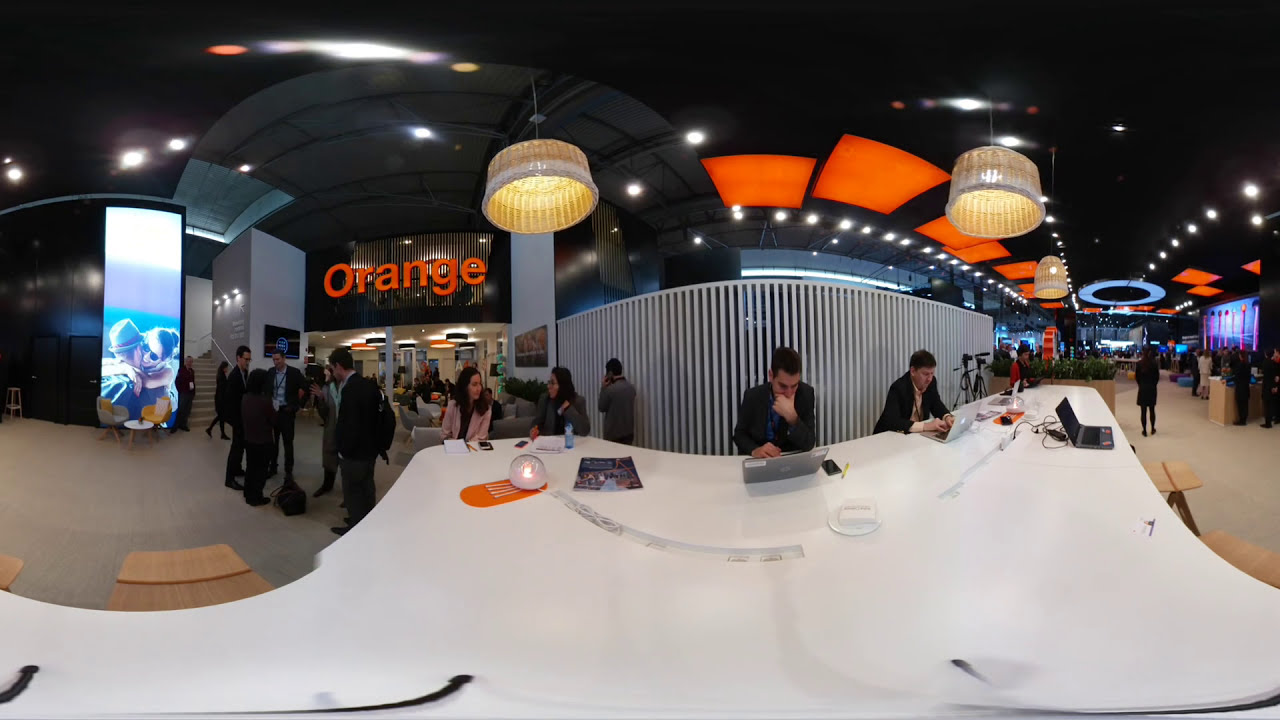This detailed, horizontal rectangular photograph, taken with an unusual lens, captures a bustling indoor congregation area, likely in a mall, exhibition, or airport. Prominently featured in the center of the image is a large, curved white table where several people, including two gentlemen with silver Apple laptops, are seated and working. Among them are also a couple of women, further adding to the busy atmosphere. Behind the table, a storefront with the word "orange" displayed in bright orange lettering stands out. The store's illuminated windows and interior lights add to the vibrancy of the setting. Additionally, the image shows several people walking around in the background, enhancing the sense of motion and activity in the space. To the left of the table, a bright screen displays an image, while overhead, bohemian-style lamps and futuristic décor contribute to the area’s modern aesthetic. On the right, a hallway extends far into the distance, suggesting the space is expansive. The dominant colors are white, black, tan, orange, gray, blue, and yellow, punctuating the lively and dynamic feel of the environment.